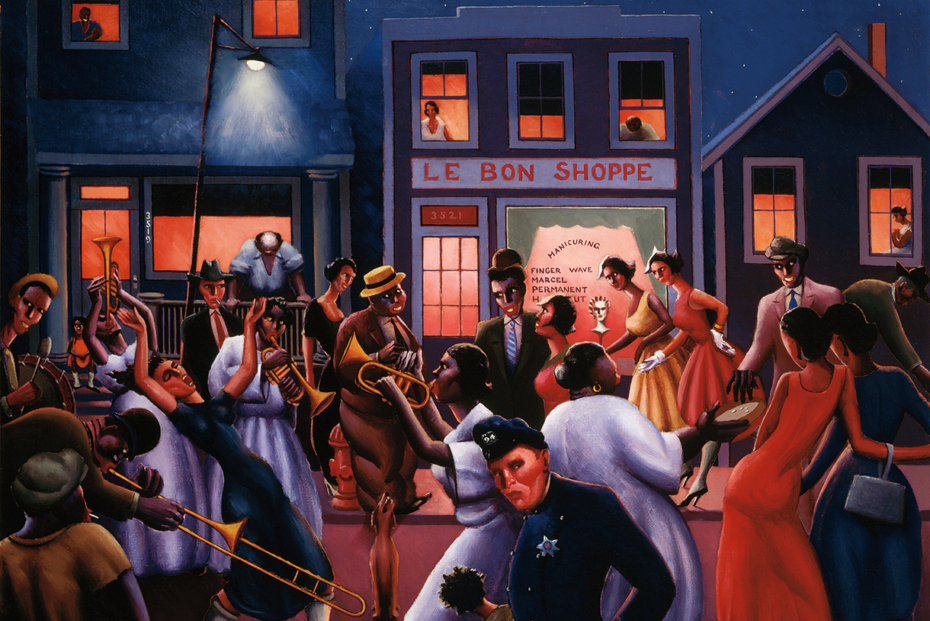The painting depicts a lively street celebration at night, bathed in the glow of a single lamppost. At the forefront stands a police officer with a star badge on his hat, who appears to be looking directly at the viewer. Beside him, a dog sits attentively. The scene is vibrant with activity; a band with various brass instruments—including trumpets, trombones, and a French horn—plays energetically on the left side, their faces filled with joy. In the center, multiple women in colorful dresses dance exuberantly; one in a white dress reaches out with a trumpet in hand toward another woman also clad in white who is gracefully spinning. There are also men in sharp suits, one notably wearing a pinkish-red suit with black gloves and a brown hat. 

Behind the crowd, three buildings rise prominently. The central building, labeled "Le Bon Shoppe," features two upper-story windows with residents peering out; one window's shade is drawn three-quarters of the way, casting a partial shadow. The shop's sign advertises "manicuring, finger wave, Marcel, permanent haircut." To its left, a residential building has a person standing on a small porch, intently observing the festivities, while another figure looks down from a second-story window. The building on the right, marked by two windows, displays a resident in one of the windows, not engaged with the bustling street below. Every character and detail in the scene contributes to the dynamic and festive atmosphere of this celebration, immortalized in an evocative, painterly style.